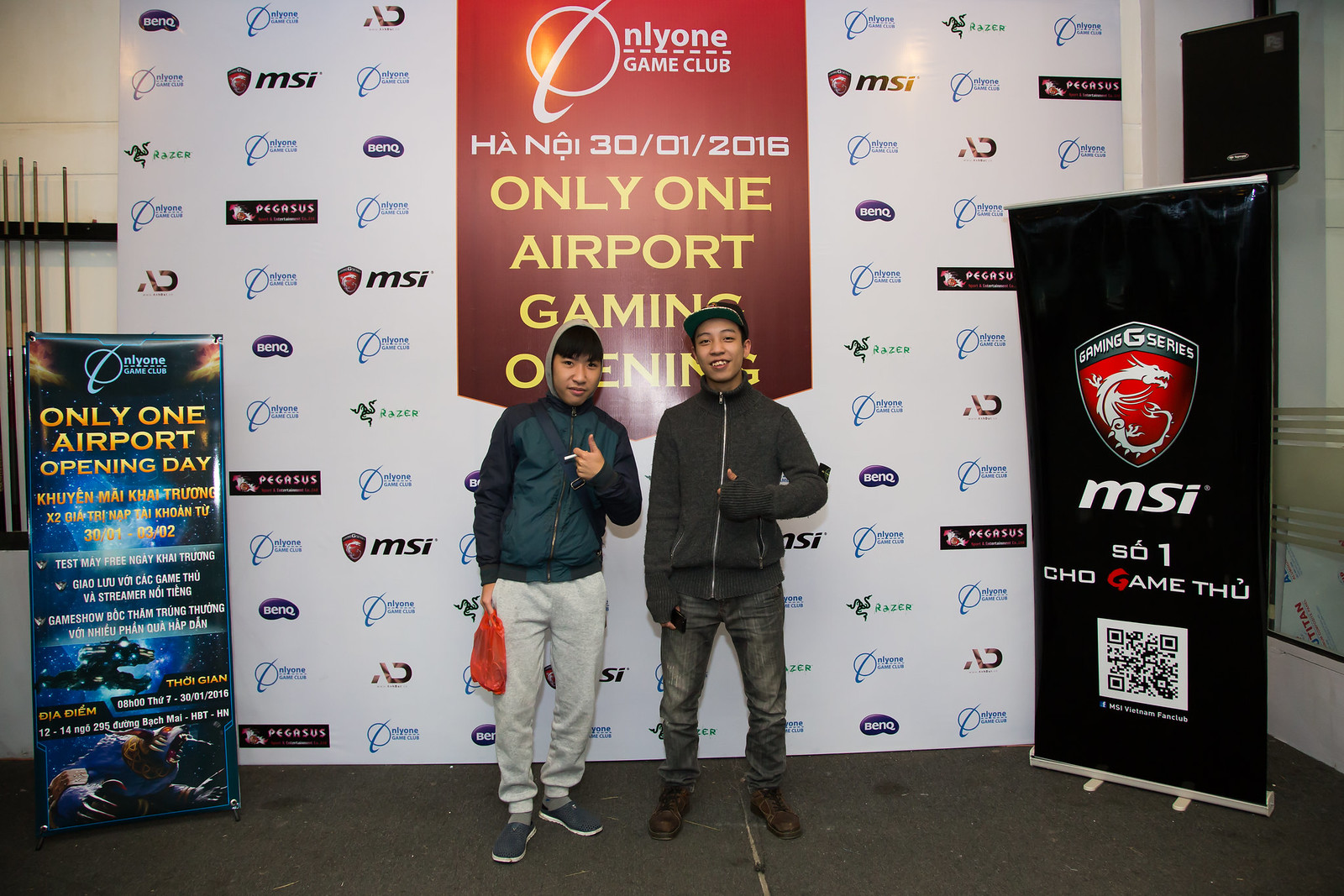In the photograph taken at a gaming event, two Asian young men pose in front of a large billboard that showcases multiple event sponsors such as Razer, MSI, and BenQ. The man on the left, who is wearing a green jacket, white sweatpants, and blue shoes, holds an orange bag. The man on the right, dressed in a gray jacket and dark gray sweatpants, is beside him. They stand before a white poster board with a prominent red banner down the middle that reads "Nylon Game Club" and "Hanoi 30-01-2016" in white font, with "Only One Airport Gaming Opening" in yellow. The billboard is a collage of logos and promotional messages, featuring MSI's black and red shield with a dragon emblem, and the text "Gaming G Series" in white on a gray background. Other brand logos such as BenQ, Razer, and Purgasus are interspersed, creating a vibrant backdrop that firmly situates the scene within the energetic milieu of a gaming event.